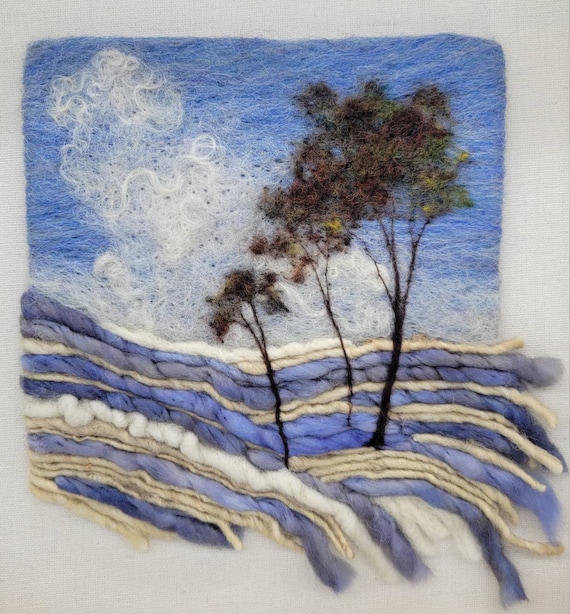This artwork portrays a detailed beach scene, meticulously crafted using various types of yarn and wool-like materials. The piece is set against a white or gray background, providing a neutral backdrop that highlights the vibrant textures and colors. The sky is created from tufted wool, giving it a fluffy appearance, with white, puffy clouds made from shredded and unraveled yarn, enhancing their soft, airy look. 

Below the sky, a layered landscape unfolds, depicting an ocean or ground cover composed of horizontally laid strands of yarn in shades of blue, cream, white, and beige. These layers are intricately arranged to mimic the rolling waves or strata of the earth, with thicker white sections interspersed among the colors.

In the foreground, three tall trees stand prominently. Their trunks and branches are fashioned from black and brown thread or yarn, which appears to be frayed, adding textural depth. The foliage of the trees is made from a mix of green, light green, and brown yarns, frayed to imitate the leaves.

Altogether, this yarn artwork captures the serene beauty of a coastal landscape, skillfully using texture and color to bring the scene to life.